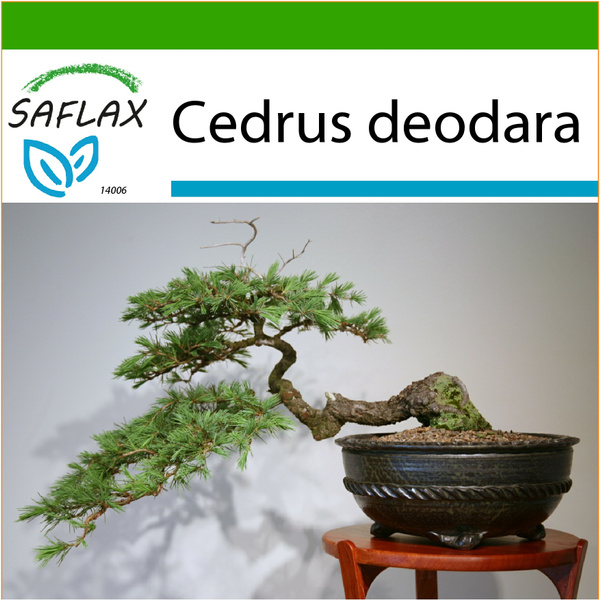The image appears to be an advertisement featuring a miniature bonsai tree, specifically identified as a Cedrus deodara. The lower three-quarters of the image showcase the bonsai tree emerging from a gray pot that sits atop a red wooden stool. The tree itself has a unique growth pattern, initially bending sharply to the left, extending downwards almost below the pot, before curving back up to display its greenery. The background is neutral white, allowing the shadow of the tree, stool, and pot to be distinctly visible against the wall.

The advertisement's top quarter features a green stripe header and contains an array of company branding elements and textual information. On the left side, there is a logo for a company named Safflax, which includes the name "Safflax" written in black font with a green chalk-like arch above it and two blue leaves beneath it. To the right of the logo is the numeric identifier "14006" in smaller black font. Beside the logo, the plant name Cedrus deodara is prominently displayed in large black letters. Beneath this text, a thin blue rectangular line separates the advertising copy from the image of the bonsai tree below.